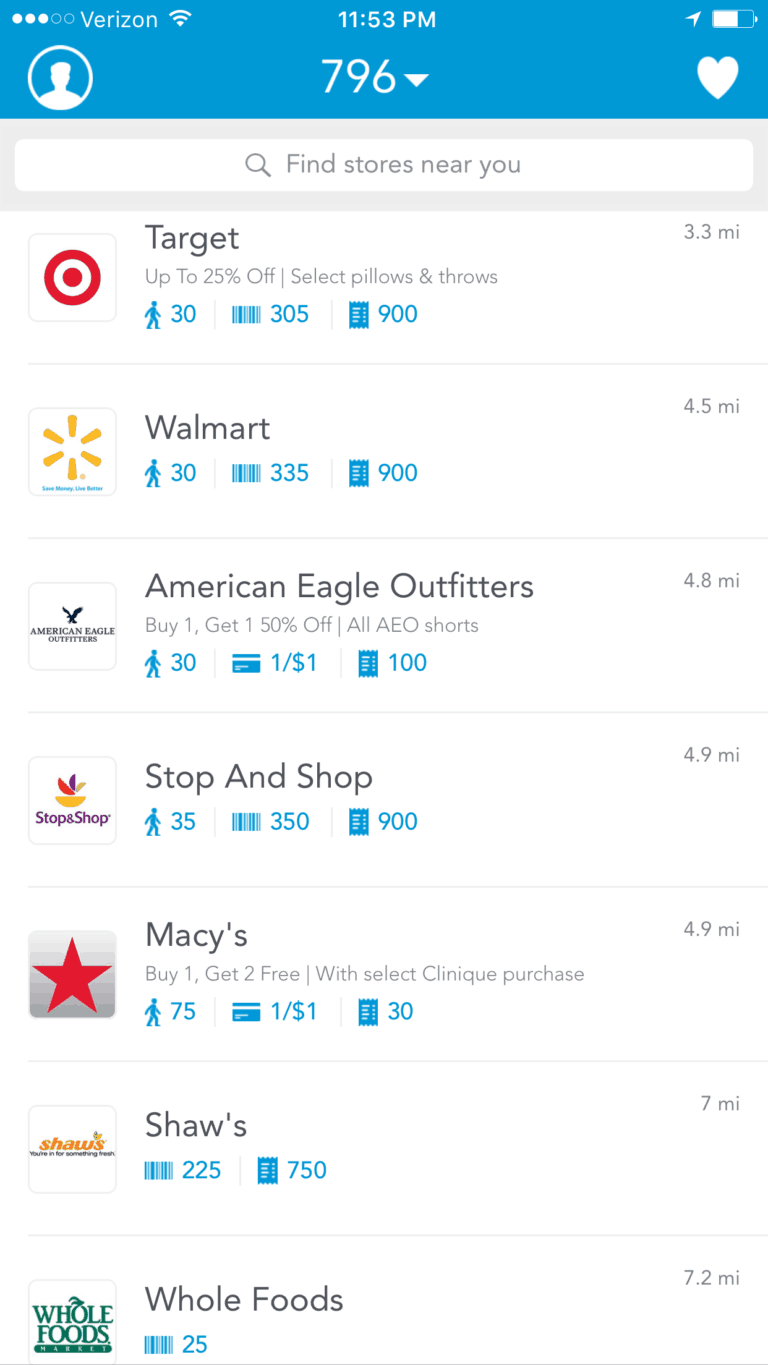This image, captured from a smartphone, showcases a mobile app screen designed to help users locate nearby stores. The top of the screen features a teal header displaying the time (11:53 PM), a heart icon, a battery life indicator, and an airplane symbol. Below this header, a search bar prompts users to "find stores near you," accompanied by a downward pointing arrow and the number 796.

The main section of the screen, set against a white background, presents a list of shopping locations with accompanying details. The first entry is for Target, featuring the store's red bullseye logo and a promotion offering up to 25% off select pillows and throws. Target is listed as 3.3 miles away. The following entry is Walmart, marked by its distinctive yellow sunburst logo, located 4.5 miles away. Next, American Eagle Outfitters is shown, represented by a box containing an eagle icon. This store is 4.8 miles away. 

Subsequent listings include Stop and Shop at 4.9 miles, Macy's at 4.9 miles, Shaw's at 7 miles, and Whole Foods at 7.2 miles, each displayed with their respective logos and distances. This well-organized layout provides a clear and concise overview of nearby shopping options and their distances from the user's location.